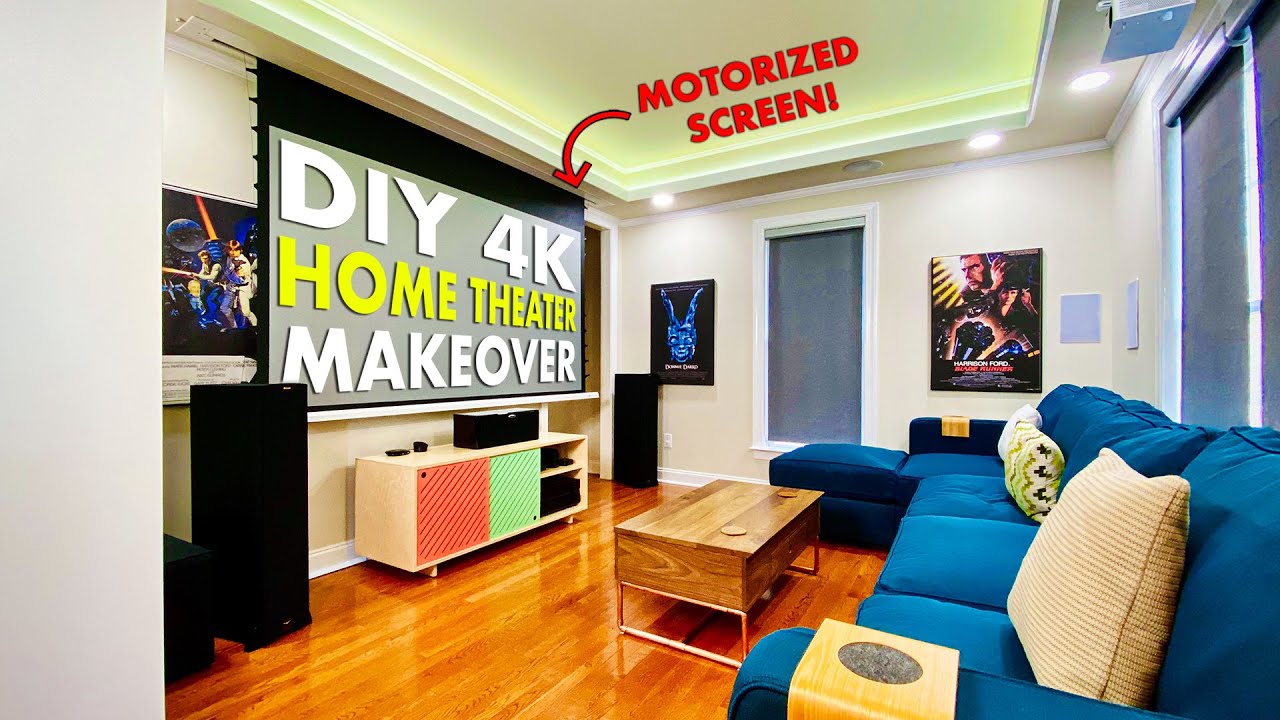The image showcases a photorealistic advertisement for a DIY 4K Home Theater Makeover, resembling a thumbnail for a YouTube video or catalog entry. Set in a stylish, modern living room, the scene features a large television screen, likely between 60 to 72 inches, displaying the text "DIY 4K Home Theater Makeover" in bold white and yellow letters. The TV is highlighted by red text at the top of the image stating "Motorized Screen" with an arrow pointing down, indicating the screen's ability to retract. The room includes a comfortable blue couch with wooden cup holders and accented throw pillows, positioned to face the TV. The space is decorated with posters, possibly rock and roll-themed, and is framed with crown molding. The mid-brown polished wooden floor complements the off-white walls, while large, stylish speakers and track lighting enhance the overall ambiance. A wooden coffee table is placed in front of the couch, adding to the cozy, yet modern feel of this home theater setup.